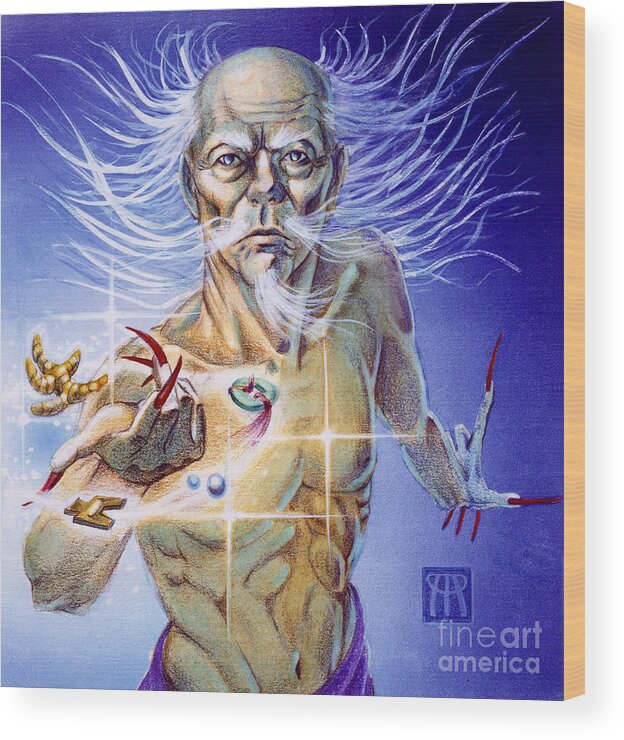This detailed artwork, likely created using colored pencils or pastels, features an elderly, mystical-looking man with a strong resemblance to Confucius or a wizard-like figure. The man exhibits a blend of serious and eerie expressions, with overgrown, dagger-like red fingernails adding to his enigmatic aura. His long, scraggly gray hair and mustache frame his balding head, while wispy, white chin hair extends downward. He is depicted bare-chested, revealing a well-defined build from head to belly button, and is draped in a purple cloth from the waist down. The background of the piece transitions through shades of blue, enhancing the ethereal feel of the scene. Intriguingly, there are elements like what appears to be ginseng or ginger root and various coins near the figure. A watermark for Fine Art America, along with the artist’s personal symbol or signature, is visible in the bottom-right corner of the canvas, further authenticating this unique piece.